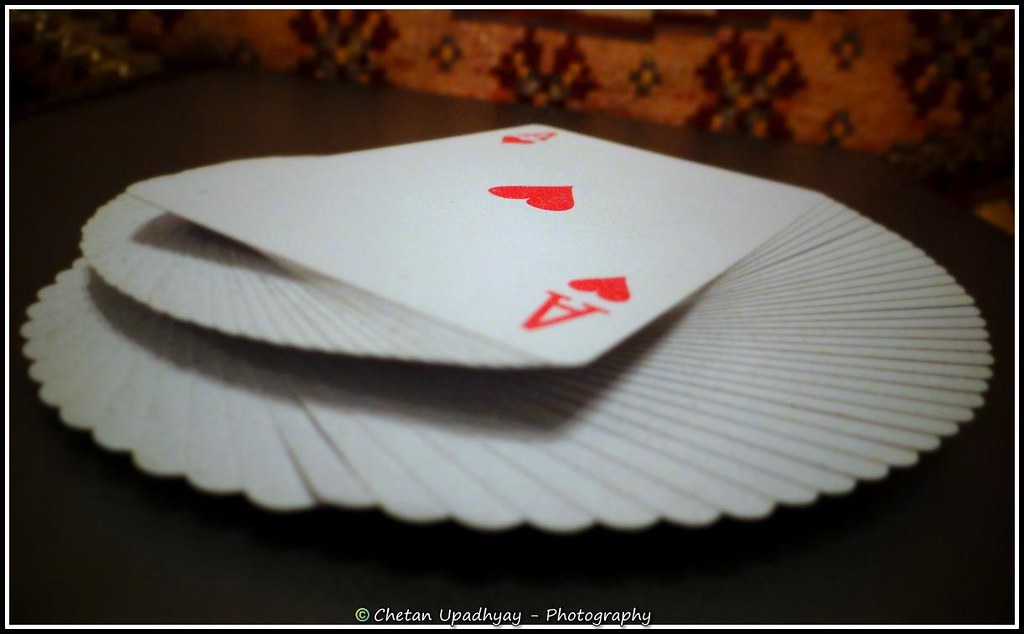The image showcases a deck of playing cards artfully arranged on a slightly dark brown table. The surface of the table appears almost black at the bottom due to shadows, but gradually lightens to a brown hue as you move outward. The background is intricately designed with decorative patterns featuring Xs, plus signs, and small flower motifs in tan, red, and green colors, though the low light obscures these details somewhat.

At the bottom center of the image, a white copyright symbol and the text "Chetan Updehay-Photography" indicate the photographer’s professional touch. 

In the center of the image, the playing cards are meticulously fanned out in a spiral pattern radiating from an eye-catching, large Ace of Hearts at the core. The card arrangement creates a circular, almost hypnotic effect, with the cards diminishing in size and overlapping each other as they extend outward, forming a harmonious blend of symmetry and elegance.